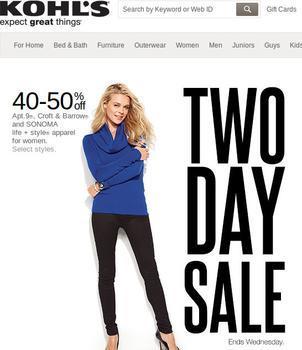The image depicts a digital interface of a Kohl's website, which could be viewed either on a mobile device or a desktop computer. The background is predominantly white. At the very top, there is a white header featuring the Kohl's logo, accompanied by the tagline "Expect Great Things." To the right of this header is a search box for site navigation.

Beneath the header lies a gray menu stripe that organizes various clothing and home categories, such as Home, Bed and Bath, Furniture, Elderware, Women, Men, Juniors, Guys, Kids. Below this menu is the main content area, also with a white background.

Dominating the main page is a bold announcement of a "Two-Day Sale." Centrally positioned on the right side of this announcement is an image of a woman wearing black leggings, high heels, and a blue sweater. To her left, the promotion details are highlighted in large text, stating a discount of "40-50% off." Beneath these promotional details is a smaller text providing a brief description of the clothing items on sale. The sale is noted to conclude on Wednesday.